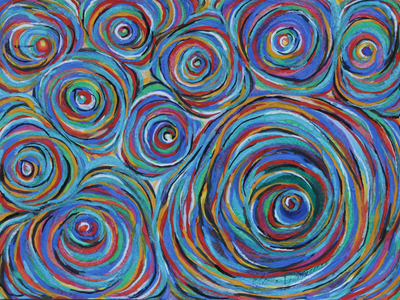This image showcases a vibrant and intricate abstract painting, possibly oil on canvas, dominated by various spiral designs that create a dynamic composition. Set within a small horizontal rectangle, the painting features numerous colorful swirls—green, blue, red, orange—emerging from central white points and expanding outward in concentric circles. The most prominent spiral occupies the bottom right corner, spanning approximately 30 to 40% of the artwork, drawing immediate attention with its large, vivid presence. Surrounding this are ten smaller spirals scattered throughout the canvas. Notably, the bottom left of the painting includes another larger-than-average spiral, while the top left houses a cluster of five spirals, with one central, larger spiral flanked by four smaller ones. Additionally, three smaller spirals trail across the top of the large bottom-right swirl, with light blue predominating the spaces between the spirals, accented by sporadic touches of orange. The overall effect is a mesmerizing, swirling tapestry of colors reminiscent of microscopic germs, all seamlessly blending into a captivating abstract design.